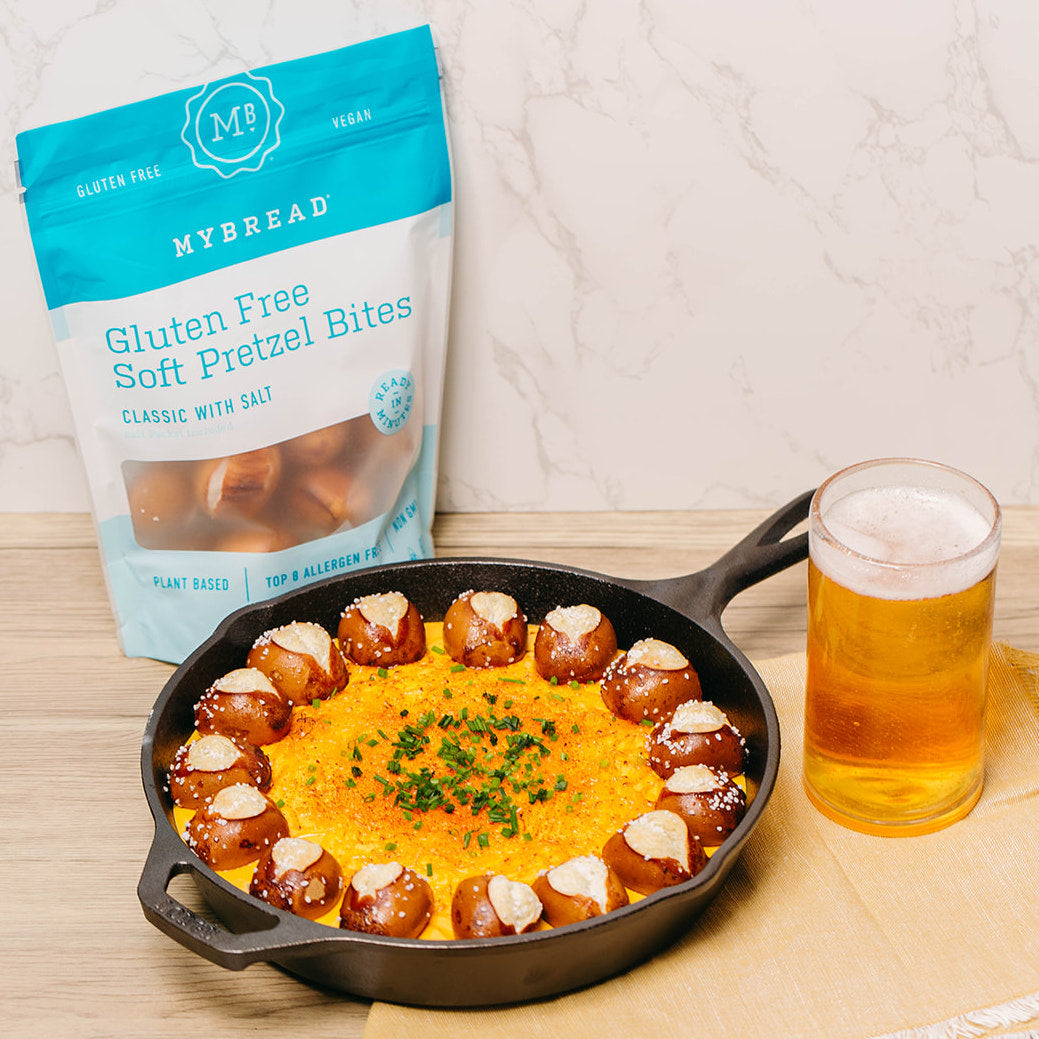In a brightly lit kitchen with a marble-patterned gray and white wall and a light wood floor, there is a close-up photo of a freshly prepared appetizer. Central to the image is a black metal skillet with a long handle positioned to the right and a smaller handle on the left. The skillet's base is filled with a vibrant yellow substance, possibly melted cheese or eggs, which creates a striking contrast with the pan. Scattered atop this yellow base are generous green garnishes, potentially onions or herbs, adding a fresh touch to the dish.

Encircling the outer edge of the skillet, neatly arranged, are golden-brown pretzel bites topped with a white substance, possibly salt. These pretzel bites are soft, with a crispy exterior, reminiscent of pretzel rolls. A glass of beer, exhibiting a rich amber color with a foamy head, is positioned to the right, next to a beige napkin. In the background, to the upper left, a blue-and-white bag labeled "gluten-free soft pretzel bites" from "My Bread" sits propped open, presenting more of the appetizing pretzel bites inside. This setting, likely a kitchen or dining room, seamlessly blends the rustic and the contemporary, highlighting the delicious, gluten-free pretzel bite dish at its center.